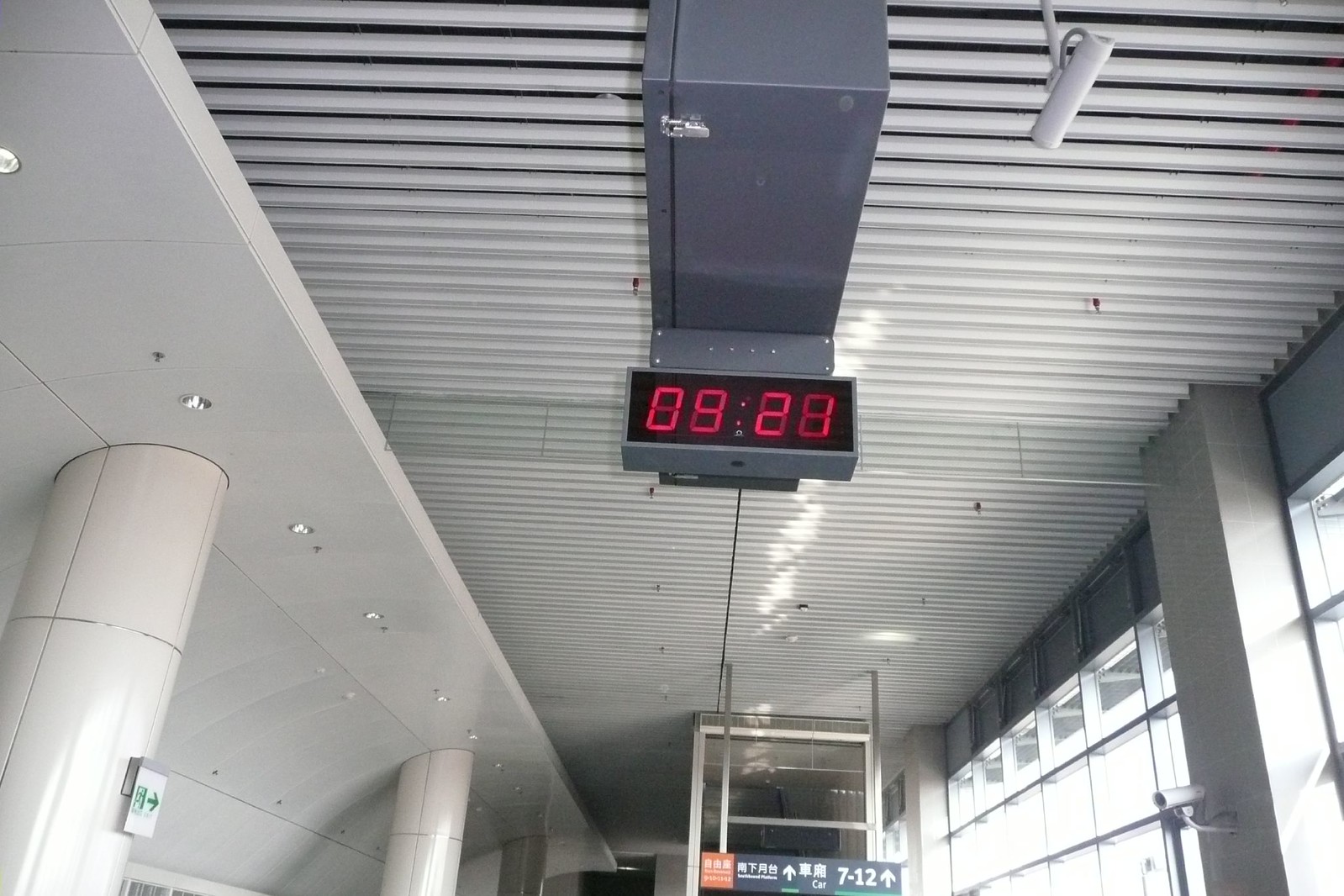The photograph, taken from an upward angle, showcases the interior of a building with a slightly wider-than-tall aspect ratio. The central focus is a digital clock mounted on the white slatted ceiling, which runs horizontally across the image. The clock hangs from a gray bracket and features a dark screen with red digits displaying "9:21". The ceiling, made of materials resembling plastic or metal blinds, spans the entire width of the image.

On the right side of the frame, there are windows formed by clear glass bricks in a grid pattern reminiscent of the Brady Bunch style, allowing light to filter through and illuminate the space. The left side features two off-white columns supporting the ceiling, which also contains circular lights. Additionally, a small black sign in the background, inscribed with "7-21" and an upward-pointing arrow in white, hints at further navigational details. A subtle hint of orange is visible in the distance, adding a slight pop of color to the predominantly white and gray interior.